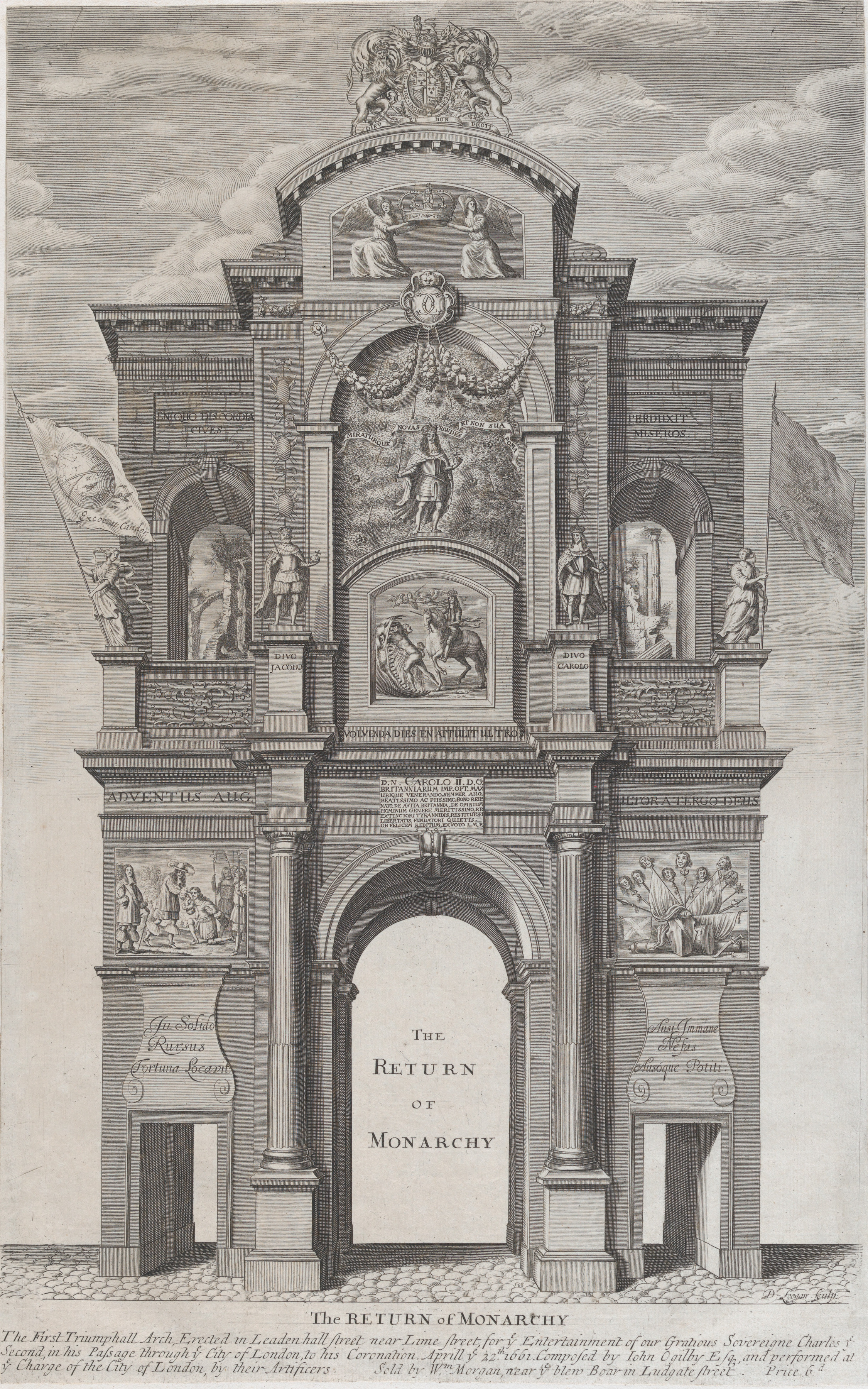The image is a detailed black and white hand-drawn etching reminiscent of an illustration from a very old book, depicting a grand, triumphal arch with Romanesque features. The large central arch, flanked by two smaller doorways with pillars, is adorned with detailed sculptures. Above the archways, the monument rises in two tiers. The second level contains inset arched areas housing sculptures, while smaller pillars at this level support additional statues. At the top of the arch, a crest is flanked by what appear to be heraldic lions or horses standing on their hind legs. Flags are present on both the right and left sides of the arch. The arch is inscribed with various intricate, yet not easily readable texts, compounded by the phrase "The Return of Monarchy" prominently displayed both beneath the central arch and at the bottom of the image. The grandeur and stylistic elements suggest a focus on historical or royal themes, capturing the essence of monumental architecture and regal symbolism.